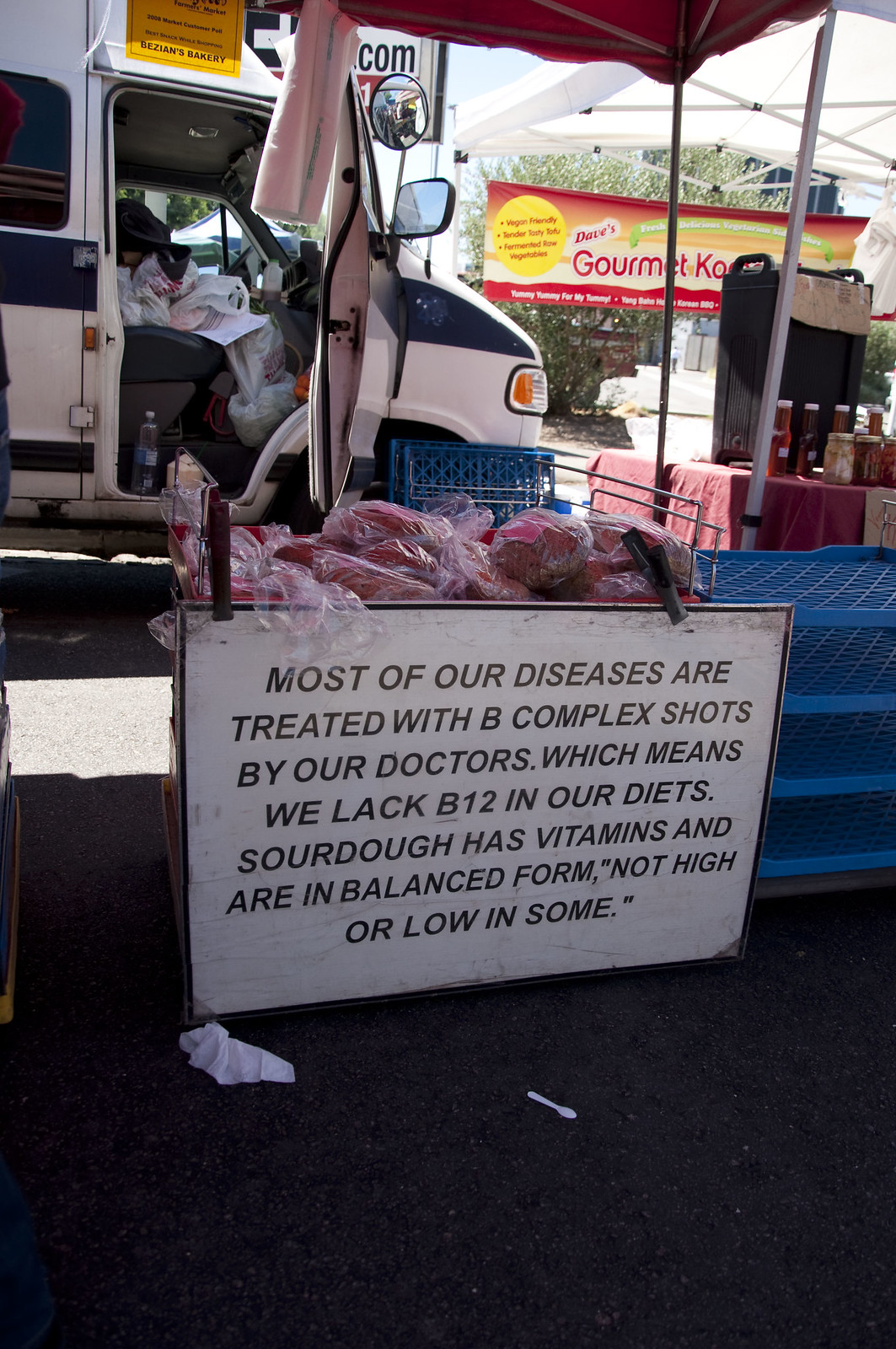The photograph depicts an outdoor scene centered around a white sign with black text that reads, "Most of our diseases are treated with B-complex shots by our doctors, which means we lack B12 in our diets. Sourdough has vitamins and are in balanced form, not high or low in some." This sign is placed in front of a table adorned with red bags and a white plastic utensil amongst other items. To the right of the image, there are blue trays and a banner with the partially visible text "Gourmet" in red. Behind the table and sign, a white RV is parked with its passenger door open, revealing a pile of white grocery bags inside. The ground in the foreground is black, scattered with a wadded-up white napkin and a white plastic spoon.